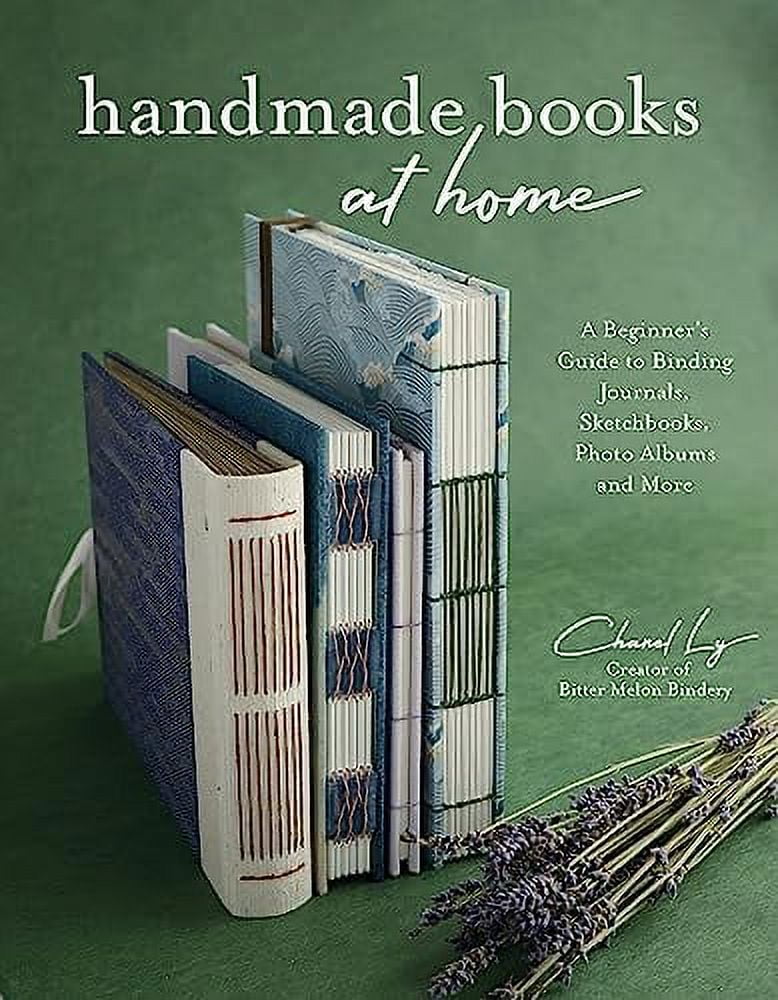The image features the cover of a book titled "Handmade Books at Home: A Beginner's Guide to Binding Journals, Sketchbooks, Photo Albums, and More," authored by Chanel Lai, the creator of Bitter Melon Bindery. The background is a uniform, greenish color, reminiscent of a backdrop used in ID photography. Prominently displayed on the cover are four handmade books of various sizes and designs, arranged in different orientations. Some books are open, allowing a peek at their interiors, while others show just their spines. The books boast vibrant, colorful designs – including blue and wavy patterns, purple with a white and red spine, and one with a brown bookmark wrapped around it. Interspersed among the books is a bouquet of dried lavender. The green background and the dried lavender sprigs provide a simple yet elegant setting that complements the artisanal nature of the books.